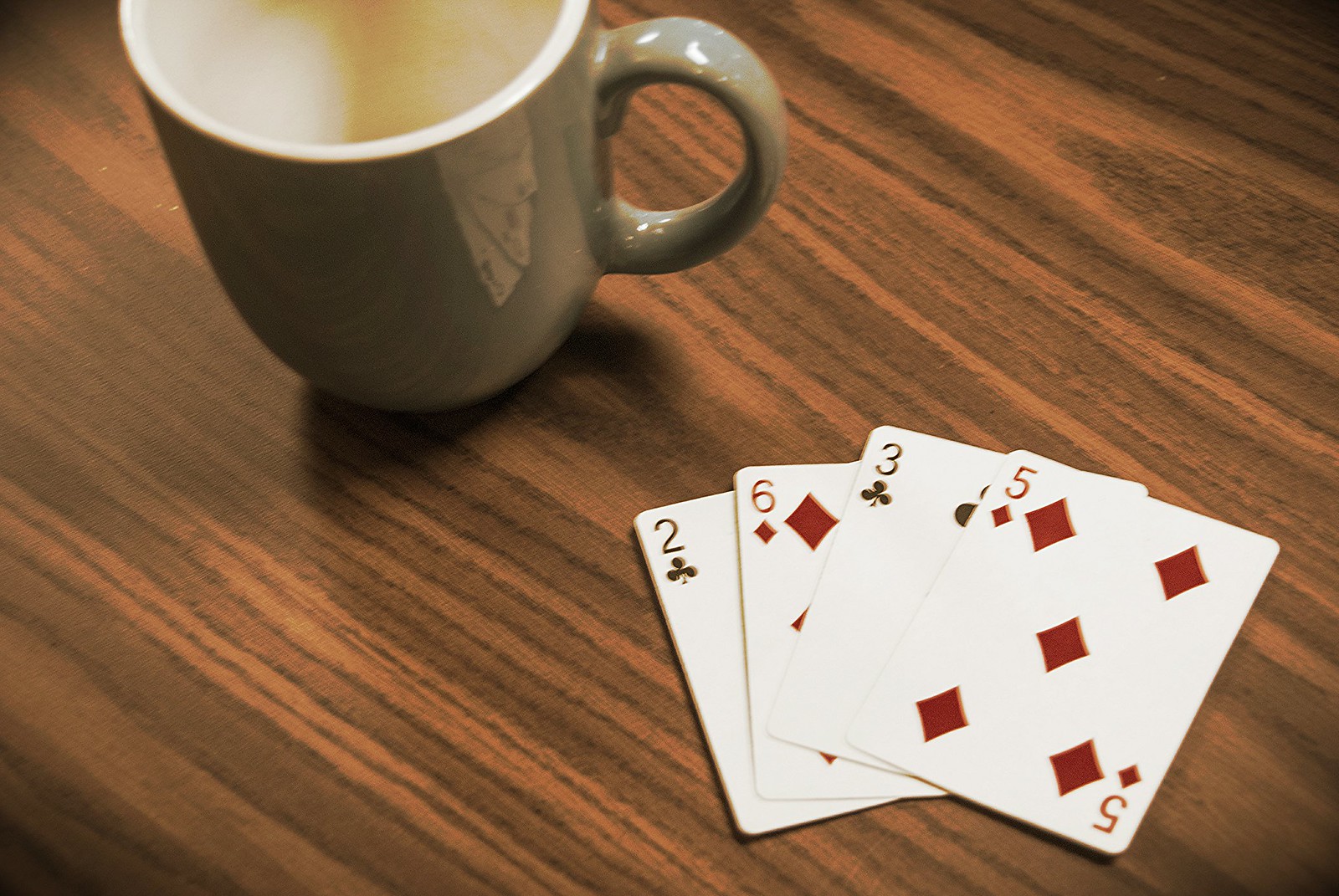This high-angle photograph captures a wooden table of dark brown hue, showcasing a close-up of its surface. On the bottom right corner of the table, there are four playing cards partially stacked but still clearly displaying their faces: the Two of Spades, Six of Diamonds, Three of Spades, and Five of Diamonds. Positioned on the top left corner of the table, a ceramic coffee mug of a grayish-blue color is casting a subtle, dark shadow. The tight framing of the image ensures that the viewer's focus remains on the playing cards and the coffee mug, with no other elements such as table legs or background visible. The overall composition emphasizes the details and textures of these few items.